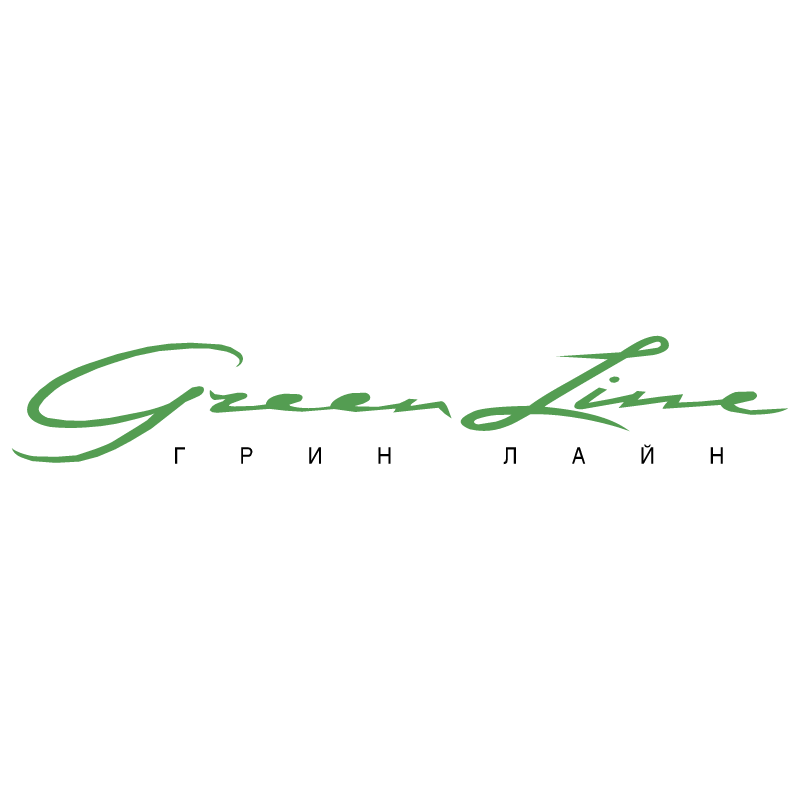The image features a logo centered on a white background, characterized by its simplicity and vibrancy. Dominating the logo is the phrase "Green Live," written in an elegant, cursive font rendered in a lively light green color. The "G" and "L" in "Green Live" are capitalized, emphasizing the brand name. Directly beneath this text, in smaller font, is a sequence of characters from a non-English language, possibly Russian or Hebrew, presented in black. The foreign text consists of distinctive characters such as an upside-down L, a P, a backwards N, an H, a musical note-like shape, an A, an upside-down N with a line above it, and another H, adding a unique international flair to the logo.